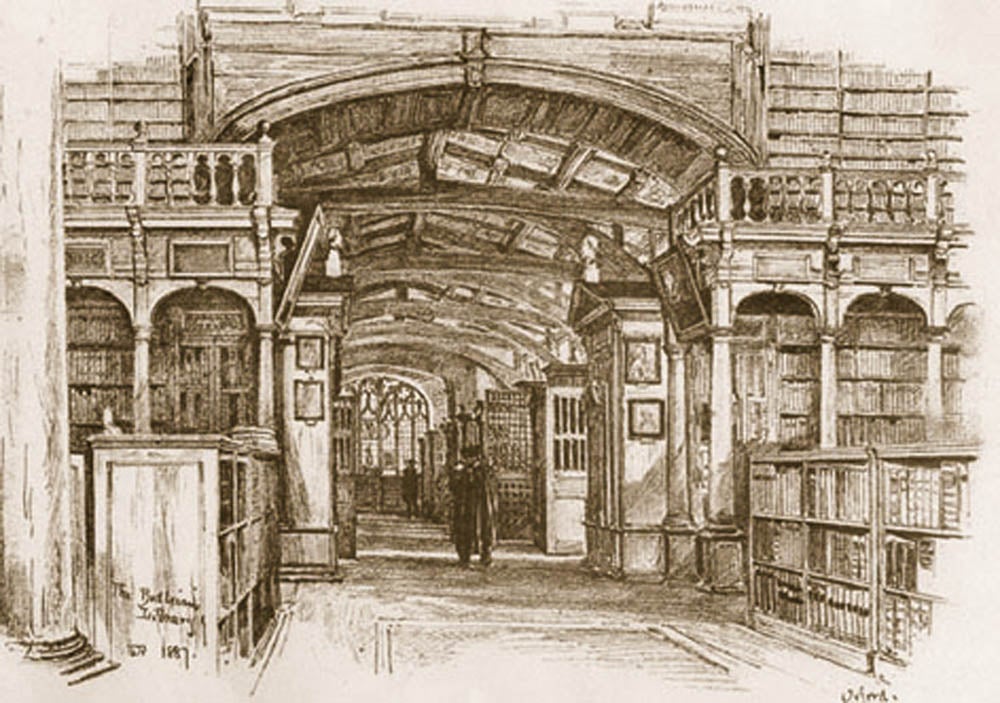This detailed pencil drawing from 1887, which appears to be titled "The Beethoven Winery," depicts the interior of an expansive, multi-level library. The perspective looks down a long hallway, with tall bookshelves lining both sides from floor to ceiling. The bookshelves are built into the structure of the building, with two levels on the walls that are accessible by a wooden balcony with classic spindles and a railing. The architectural design is detailed, showcasing wooden beam roofing and intricate column work.

The artwork reveals a wooden-floored corridor with people dressed in black garments walking in the distance. On the right side of the hallway, an open door leads into another room, and several windows can be seen at the far end, letting in light. A notable feature on the left is a white pillar, adding to the classical feel of the interior. The image is primarily composed of white, brown, and a few black accents, enhancing its vintage appeal. Through the meticulous sketching, the library’s grand yet scholarly atmosphere is vividly captured.